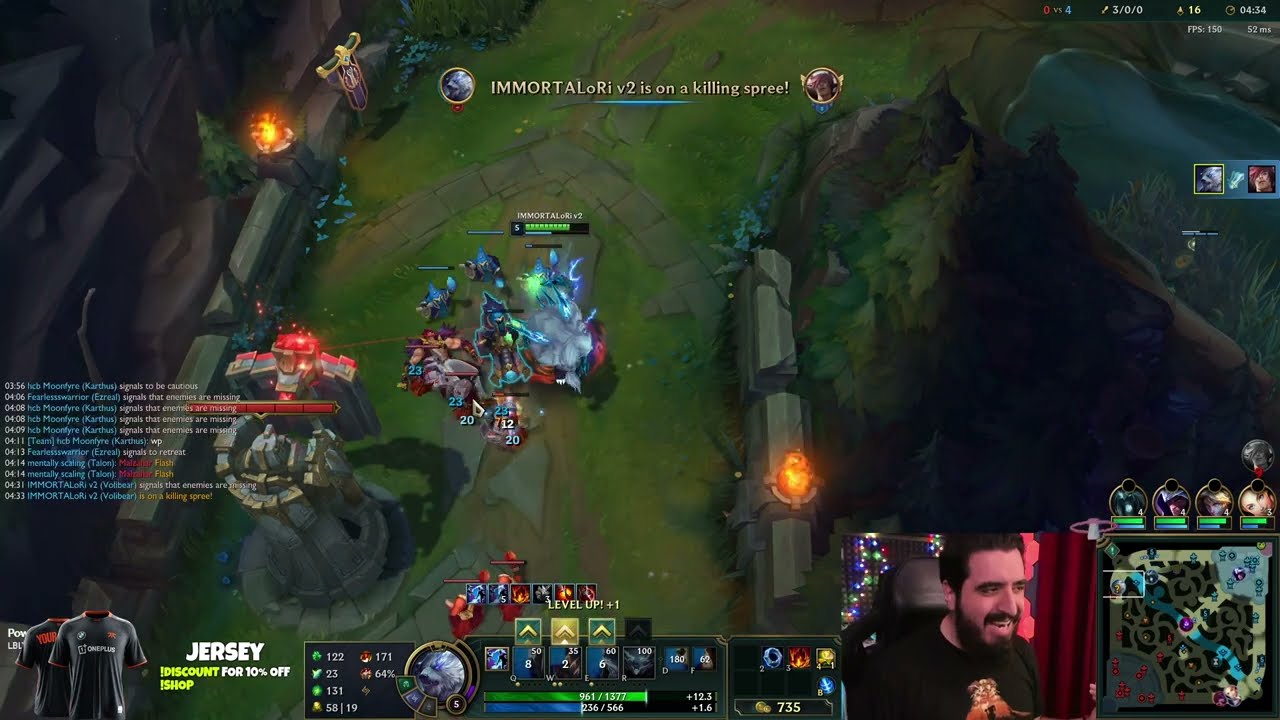The image captures a screencast of a video game being live-streamed by a bearded male streamer with slicked-back, black hair, and a black shirt featuring a gold graphic. The game appears to be an action role-playing or war game, possibly resembling League of Legends, featuring multiple characters, including monsters, engaged in combat on a path illuminated by torches. Visible game elements include damage indicators, a red glowing tower seemingly ready to attack, and explosive visuals. Also noticeable are a chat box on the left, a mini-map in the lower right, and pictures of jerseys accompanied by a 10% discount advertisement on the bottom left. The streamer, whose image appears superimposed near the mini-map, seems to be enjoying the game, as evidenced by his laughter. The background of his streaming area is marked by a red curtain.